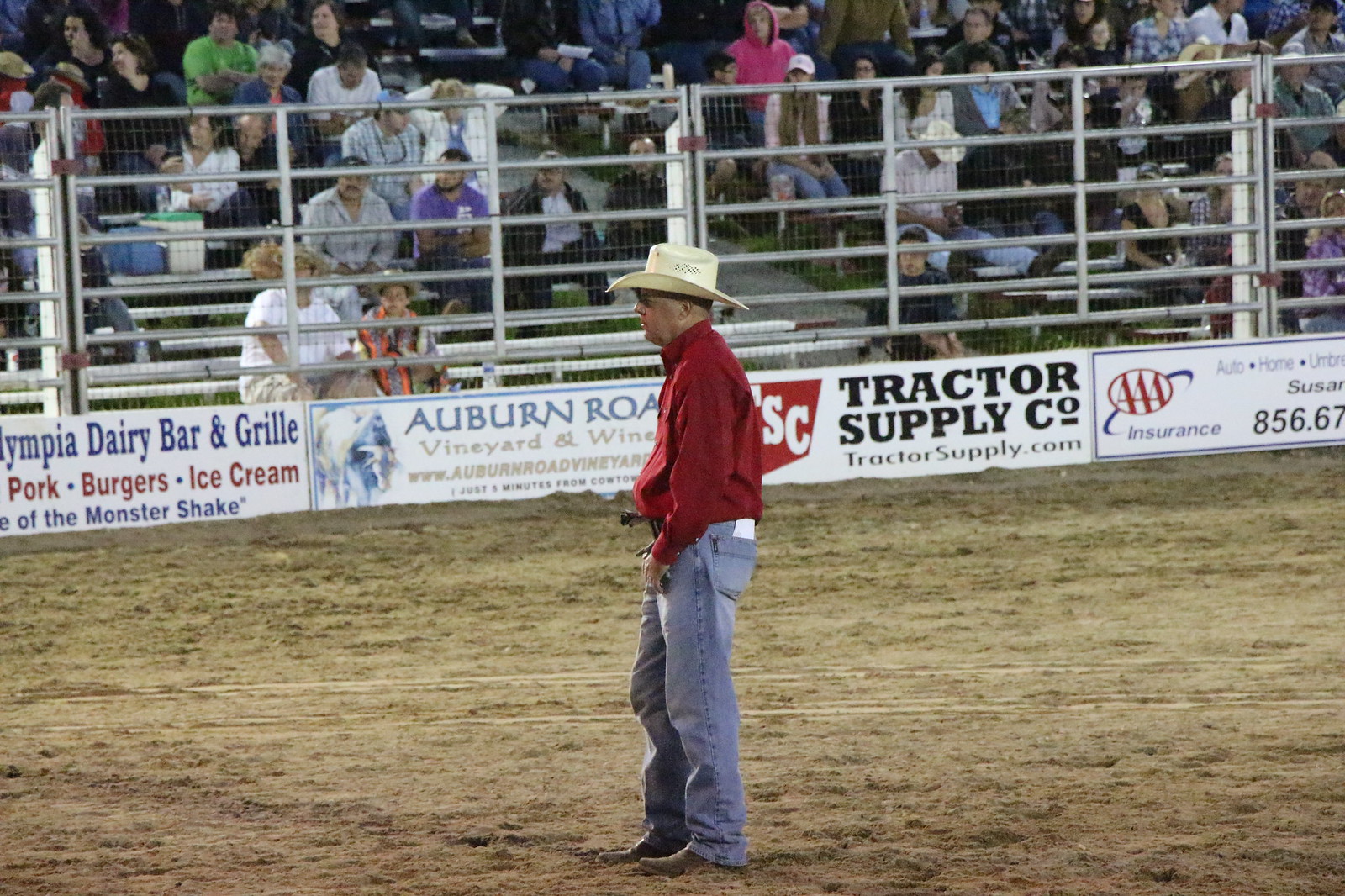In this image, we see a man dressed in blue jeans and a reddish long-sleeve shirt, wearing a cowboy hat. He stands in a grassy area that appears to be dry and brown, resembling hay. Surrounding him is a gated enclosure with an audience seated behind the gate. Along the wall beneath the gate, various signs are displayed, featuring logos and names such as Tractor Supply and AAA, likely indicating event sponsors. The setting has all the typical elements of a rodeo, with the man standing as though preparing for or participating in the event's activities.